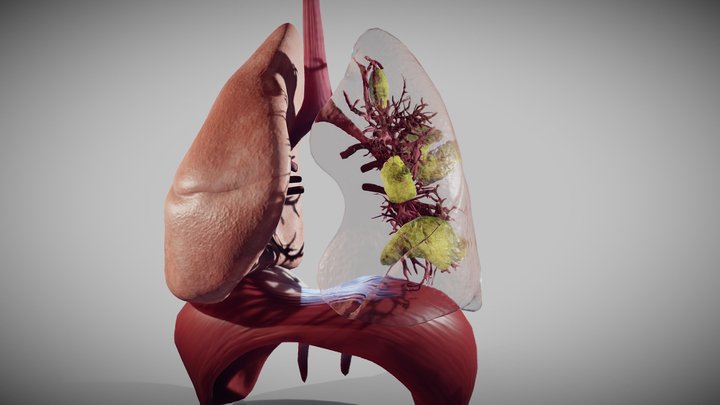This is an image of a detailed 3D model of the human respiratory system. The background features a gray gradient, darkening towards the edges. The model prominently displays the lungs and diaphragm. On the left, the lung is opaque and pink, showing the external lung tissue. The right lung is transparent, revealing intricate bronchial tubes and green blobs that possibly represent mucus or other forms. At the top, a large red blood vessel runs from the throat and branches out into both lungs. Beneath the lungs, the pink diaphragm muscle is visible, extending across the bottom with two small offshoots. The model appears shiny, indicative of a plastic or sculpture-like material, and serves as a medical representation with no text accompanying it.